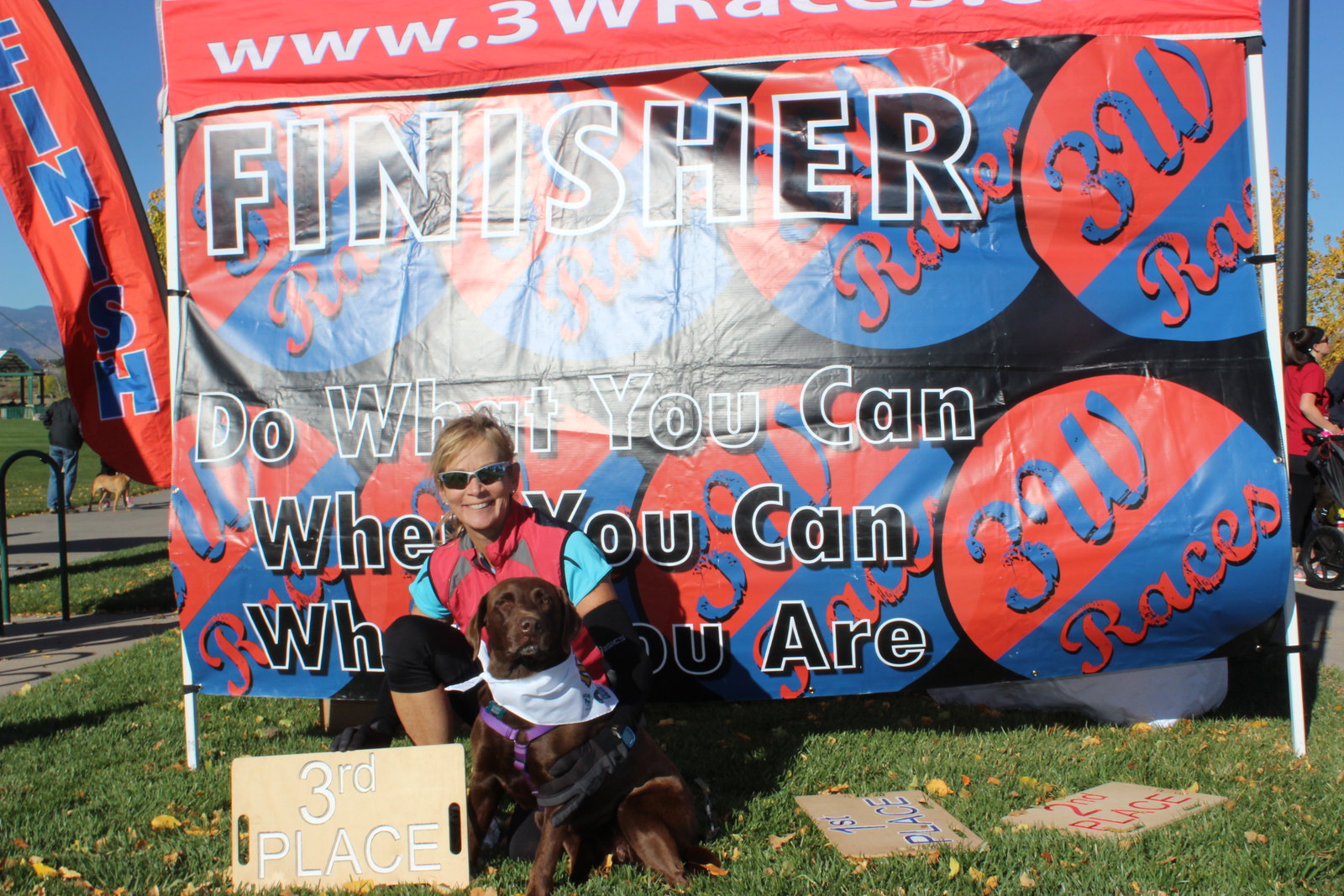In this vibrant outdoor scene, a woman is kneeling on a grassy field with her large brown Labrador Retriever, which is adorned with a white bandana and a purple harness. She is dressed in a sporty red and blue vest, black gloves, and sunglasses, indicating an athletic event. A wooden plaque in front of her proudly announces their third place finish. To the side, first and second place plaques lie discarded on the grass. Dominating the backdrop is a colorful promotional banner in shades of black, red, and blue, emblazoned with the motivational phrase: "Finisher, do what you can when you can, where you are." In the background, a smattering of other participants with their dogs is visible, enhancing the lively atmosphere of this dog-inclusive sporting event.